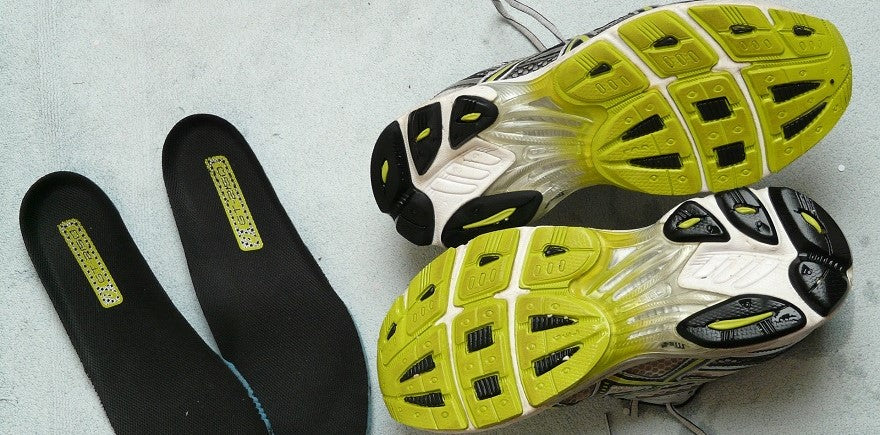The image depicts a detailed scene of a pair of sneakers and their insoles displayed on a gray surface. On the left side, the insoles have been removed from the shoes and positioned side by side; they are predominantly black with a yellow label on the heel section. On the right side of the image, the sneakers are shown upside down, displaying their soles. The shoes feature a complex color pattern: the area towards the toes is yellow, the midsection is gray, and the heel area is white with five black cushioning pads. The sneakers also have visible gray shoelaces and lime green accents on the upper part, interspersed with white lines. Additionally, there is noticeable wear on the insoles, particularly on the inner part near the big toe, indicating significant usage.